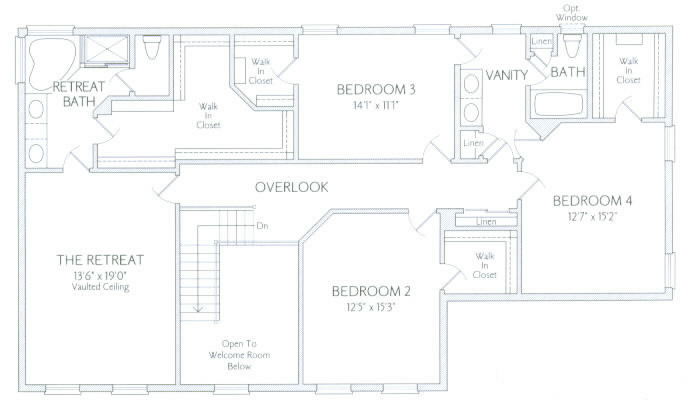This detailed floor plan, drawn in blue ink, showcases an intricately designed space providing various luxurious features. In the upper left corner, you'll find the 'Retreat Bath,' featuring a spacious whirlpool tub, a toilet, and a double sink vanity, which seamlessly connects to a large walk-in closet. Moving from the closet, you enter a 'Retreat' area that measures 13.6 by 19 feet and boasts a vaulted ceiling. Through the adjoining door, you encounter an overlook and stairway that opens up to a welcoming room below. 

Adjacent to this space is Bedroom Number Two, which measures 12.5 by 15.3 feet and includes a sizable walk-in closet. Following the hallway from this bedroom, you pass a convenient linen closet before reaching Bedroom Three on the opposite side. This bedroom measures 14.1 by 11.1 feet and also features a large walk-in closet. Continuing down the hallway, you find a well-appointed bathroom complete with a spacious double vanity, a bath, a toilet, and another linen closet. Finally, positioned at the back side of this level is another generous walk-in closet and Bedroom Number Four. This meticulously designed layout ensures ample space and functionality throughout.